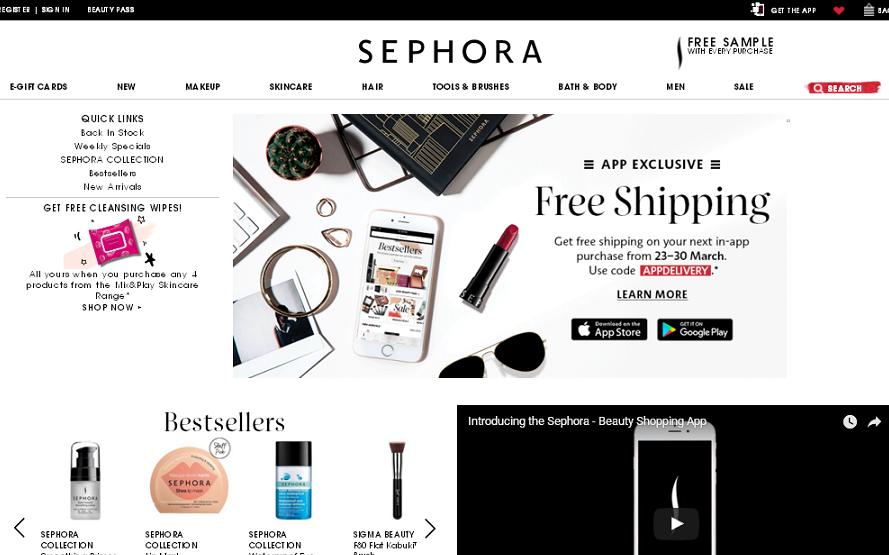This image is a screenshot of a page from the Sephora website, known for its extensive range of makeup and facial care products. The layout is predominantly black, providing a striking contrast that allows white text to stand out clearly. 

At the top of the page, there is a long, slim black rectangle featuring clickable menu items that guide visitors to different sections of the website. These items include options for "Gift Cards," "New," "Makeup," "Skincare," "Hair," "Tools & Brushes," "Bath & Body," "Men," and "Sale." Adjacent to these menu items, a red search icon allows users to easily find specific products.

Beneath this initial navigational bar, the background remains primarily black. Towards the bottom right corner, there is a video window embedded within the black background. The contrast in colors between the black background and white text highlights important promotional messages. One such message informs visitors that they will receive a free sample with every purchase. Additionally, there is an announcement about free shipping for in-app purchases made between March 23rd and 30th, using the code "appdelivery."

Scattered across the page are various images related to makeup and skincare products, enhancing the visual appeal and providing users with a glimpse of what Sephora has to offer.